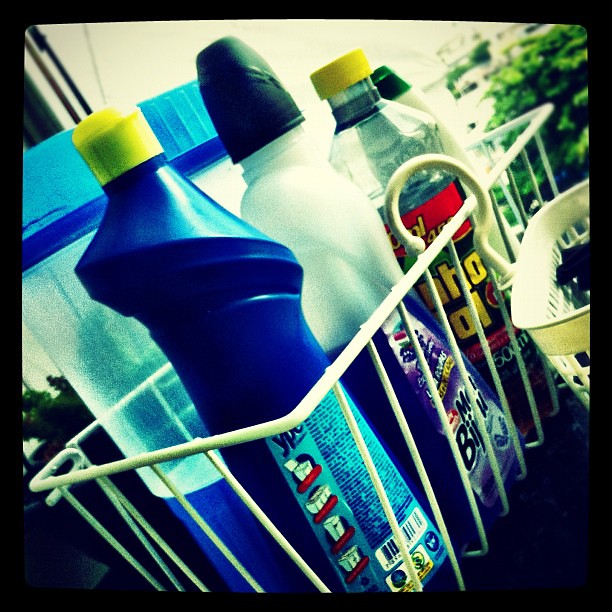The photograph features a white wire basket with vertical metal bars, holding various cleaning supplies. Positioned at an angle, the basket reveals a clear pitcher with blue liquid and a light blue oval-shaped top in the back. In the front, there's a blue bottle with a yellow lid, a white bottle with a green lid, and a clear bottle with a yellow lid, wrapped in a red advertisement with yellow writing. Additionally, a purple cleaning agent and possibly a dish soap or spray cleaner can be seen. Hanging from the right side of the basket is a white hook, and next to it is another basket with small square cutouts. A green plant is visible in the top right corner, adding a touch of nature to the scene.